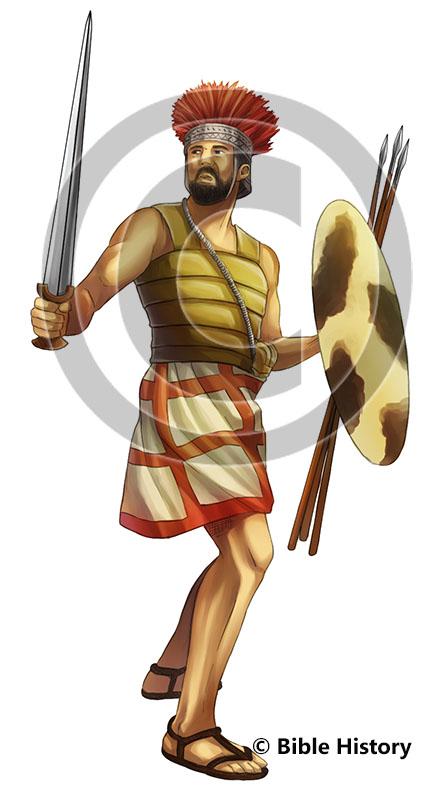The image depicts a detailed digital rendering of an ancient Roman soldier, poised for battle. He has a beige-tan complexion with a prominent brown beard and piercing brown eyes. His head is adorned with a silver headdress featuring a metal band and back, from which thin red feathers rise. The soldier's right hand grips a wide, brown-handled sword that narrows to a fine tip, while his left hand holds three wooden spears tipped with silver and an oval-shaped shield adorned with faded brown watercolor spots. His torso is encased in a leather and bronze armor resembling thick, gold bands without sleeves, exposing his muscular arms. Below, a skirt-like garment with a red grid pattern and white insets covers him, resembling a toga. His bare legs reveal musculature, leading down to dark brown sandals. The image bears a gray, opaque watermark shaped like a copyright symbol, and at the bottom, black text reading "Bible History".